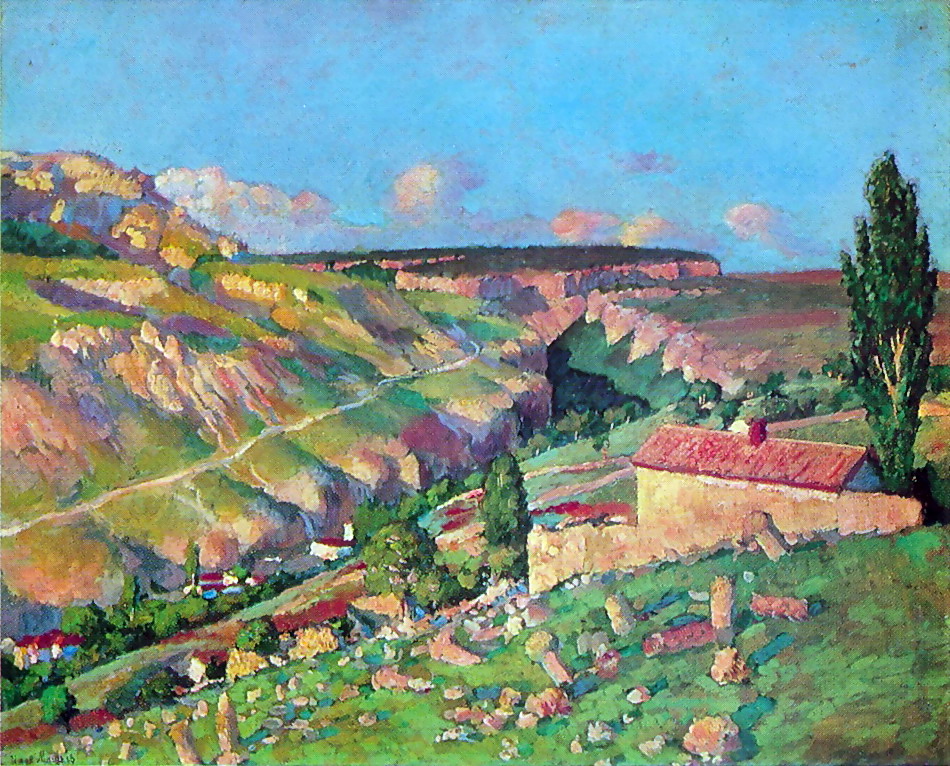This vibrant painting offers a stunning view of a quaint town nestled amidst lush, hilly landscapes. The sky is a mesmerizing mix of turquoise, blue, and hints of green and purple, interspersed with soft white and pink clouds. The left side of the artwork is dominated by bright, vibrant green fields, while the right side features slightly darker shades of green, merging into a scene of rolling hills and colorful gardens.

A prominent tree, deep green in color, stands tall on the right side of the painting. Below it, in the lower right corner, lies a charming house with a red roof and chimney, the exterior painted in a mix of cream and brownish hues. This house is surrounded by vivid flowers, possibly some mushrooms, and lush grass in its small garden.

Scattered throughout the scene are additional small houses with red roofs, set against a backdrop of a narrow meadow nestled between canyon-like walls, tinged with pink. As you gaze deeper into the painting, more plateaus, and flat areas appear, adding depth to the scenery.

Overall, the predominantly green landscape, punctuated by colorful roofs and natural features, creates a serene and picturesque panorama that captures the essence of a serene countryside town.